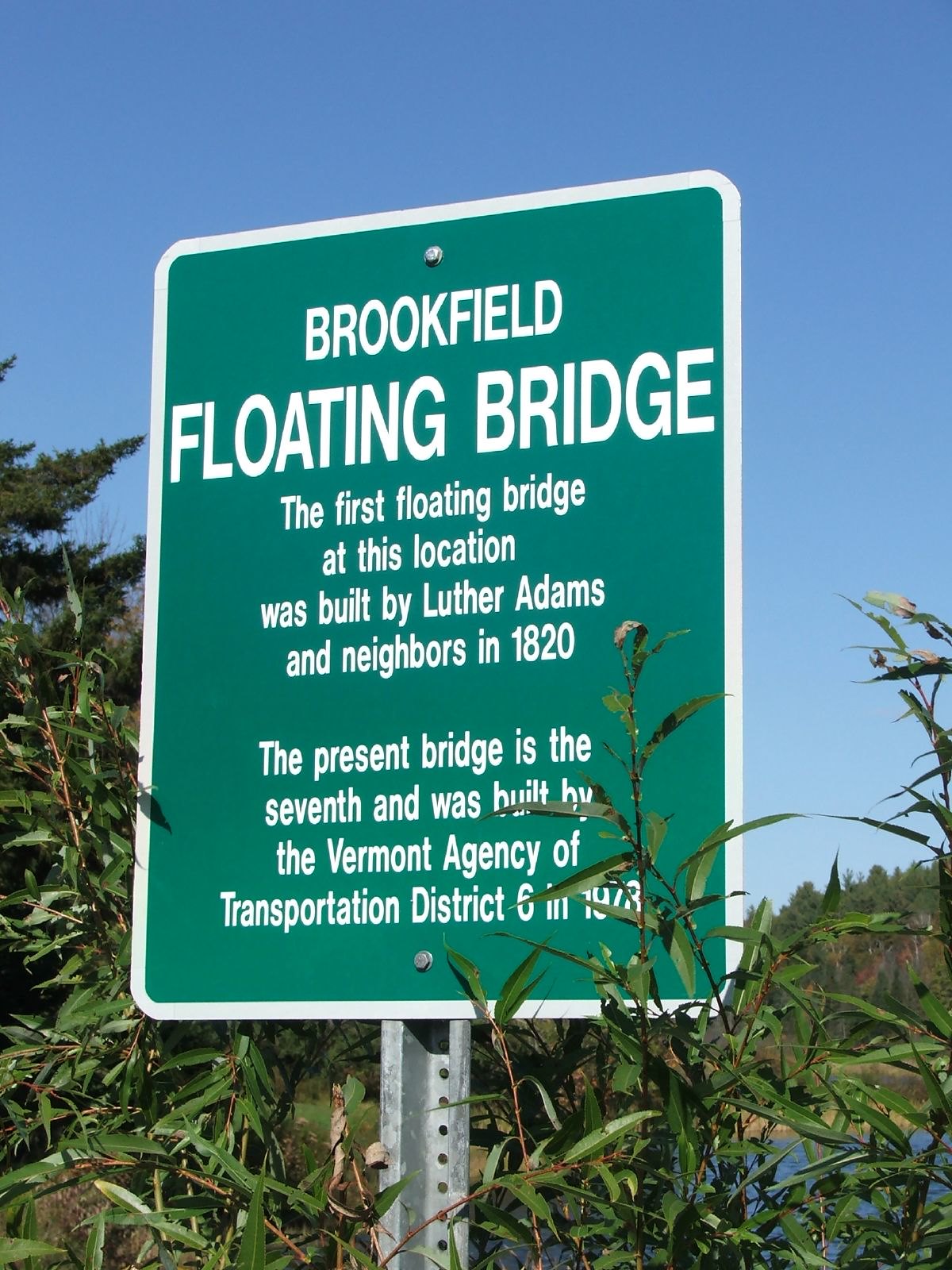A green roadside sign with white text stands on a silver-colored, hole-punched metal pole among lush green-leafed and long-leafed bushes, partially obscuring it. The sign reads: "Brookfield Floating Bridge. The first floating bridge at this location was built by Luther Adams and neighbors in 1820. The present bridge is the seventh and was built by the Vermont Agency of Transportation, District 6 in 1978." The rectangular sign is positioned among shrubs and is surrounded by large pine trees, a marsh, and visible water in the background. The image was taken outdoors during the daytime under a clear, blue sky with abundant natural light.